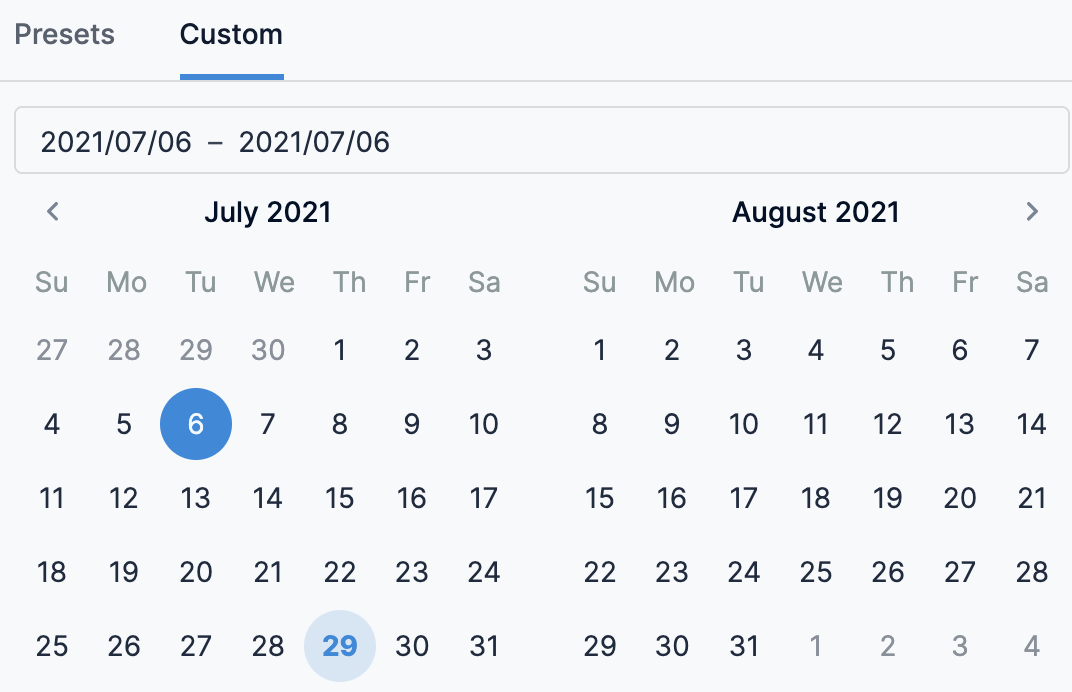The image is a screenshot of a calendar interface, with a predominantly light gray landscape layout. In the top left corner, there are two tab options: "Presets," which is in a medium gray font, and "Custom," in black font with a blue underline indicating it is the selected option. Below these tabs, a thin gray line extends horizontally across the image.

Underneath the line is a light gray, long rectangular box with subtly rounded edges and a thin gray outline, displaying the date range "2021/07/06 to 2021/07/06." Below this, two monthly calendars for July 2021 and August 2021 are displayed side by side. The months and years at the top of each calendar are bolded. The days of the week are abbreviated with "S," "M," "T," "W," "T," "F," "S," and placed at the top of each calendar.

In the calendar for July 2021, the month starts on a Thursday, while the calendar for August 2021 starts on a Sunday.